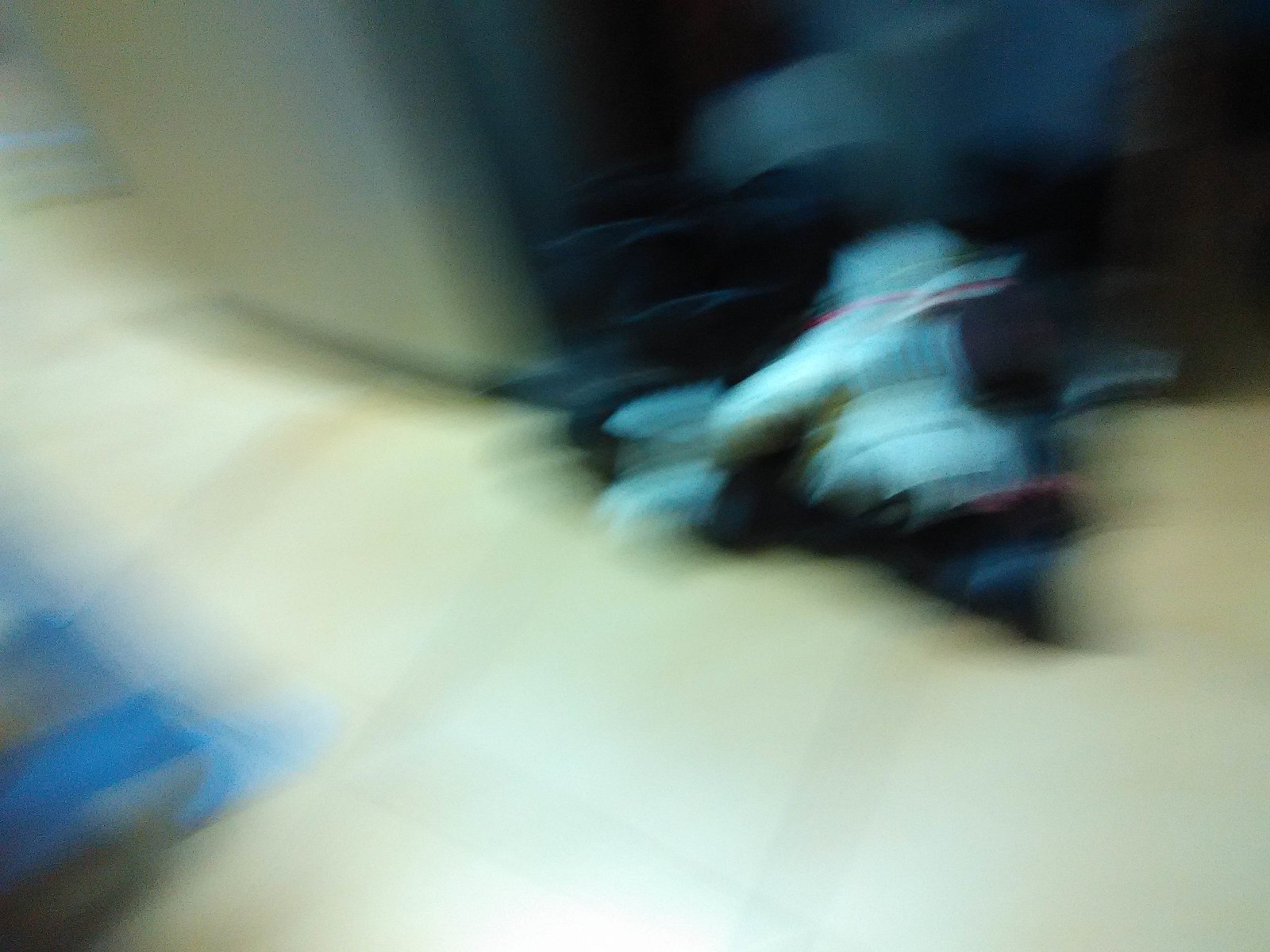This is an extremely blurry photograph with a multitude of indistinct elements, making it challenging to decipher the scene accurately. Dominating the upper half of the image is what seems to be a person, whose exact identity and activity remain unclear. This person appears to be dressed in a white outfit, possibly a coat, and seems to be seated against a backdrop that might include a wall or desk. Surrounding this figure are various indistinguishable objects, including some black and white items near what could be their face, perhaps indicating they are seated on a couch or similar piece of furniture. To the bottom left, there's a bright blue object that looks like it's made from plastic. Additionally, the scene is filled with a mixture of colors—orange, dark blue, navy blue, white, and red—suggesting other scattered items or a patterned backdrop. The floor or ground appears to be either concrete or covered in a cream-colored carpet. Specifics like a possible metal desk chair and perhaps a motorcycle add to the ambiguity of the environment.